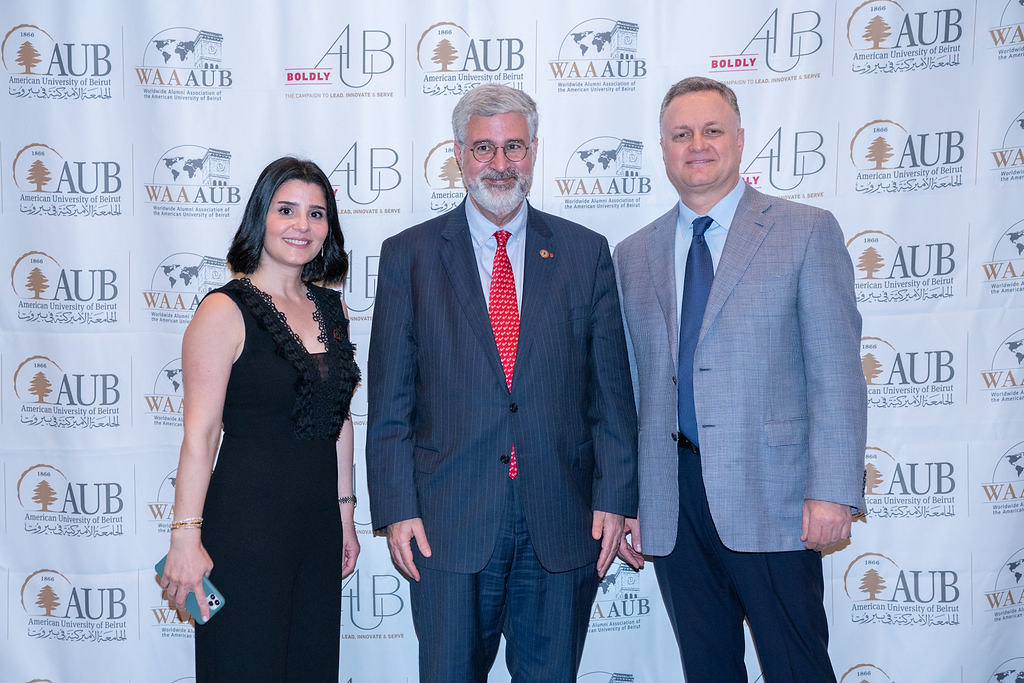In this photograph, three individuals are posing against a backdrop covered with various advertisement logos, including "AUB," "WWAUB," and "American University of Beirut." On the left stands a younger woman with a black bob haircut, dressed in an elegant black dress with a frilled collar. She holds an iPhone in her hand. In the middle is an older man, indicated by his silver hair and beard, wearing circular glasses, a navy pinstripe suit paired with a white shirt, a red tie with white dots, and dark blue pants. He is smiling warmly. To the right is another man with graying hair, dressed in a light blue shirt, a gray sports coat, a blue tie, and dark blue pants. He, too, offers a slight smile. The setting resembles a "step-and-repeat" backdrop, often used for formal events like red carpets.